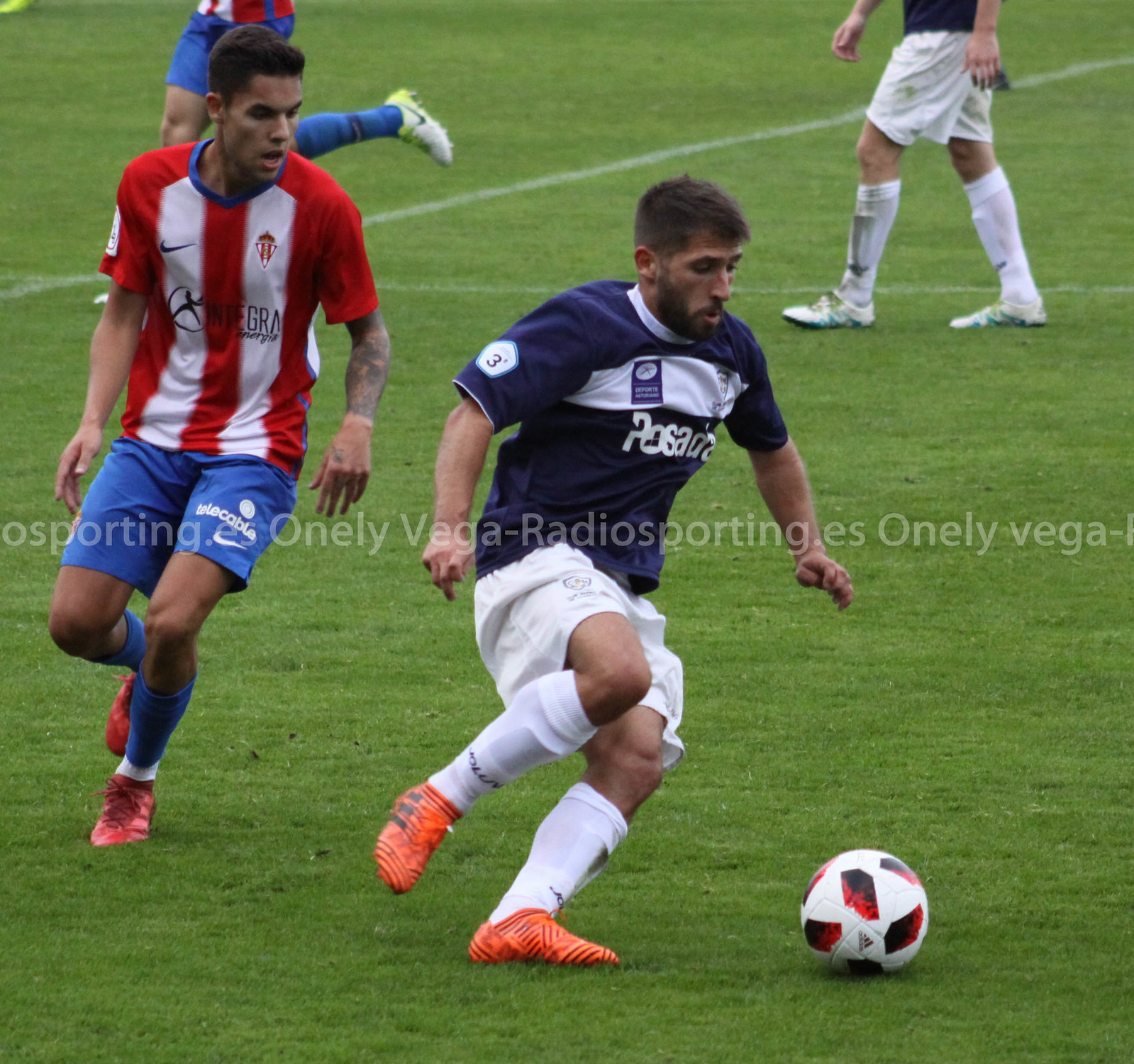In an overcast scene of a spirited soccer match, two teams—one clad in blue and another in red and white stripes—chase a soccer ball across a field marked with white chalk lines. At the center of the photograph, a player in a dark purple shirt with a large white stripe across the chest and the word "POSADA," partially visible, is about to kick the ball. He stands poised on one foot, wearing white shorts, knee-high white socks, and orange trainers. Nearby, an opponent in a red and white vertically striped shirt and blue shorts gives chase, his heavily tattooed left arm visible. Behind them, two other players, partially cropped out of the shot, can be seen running. Overlaid repeatedly across the center of the image is the text "Wanley Vega Radio Sporting.es," though it is cropped at the edges.